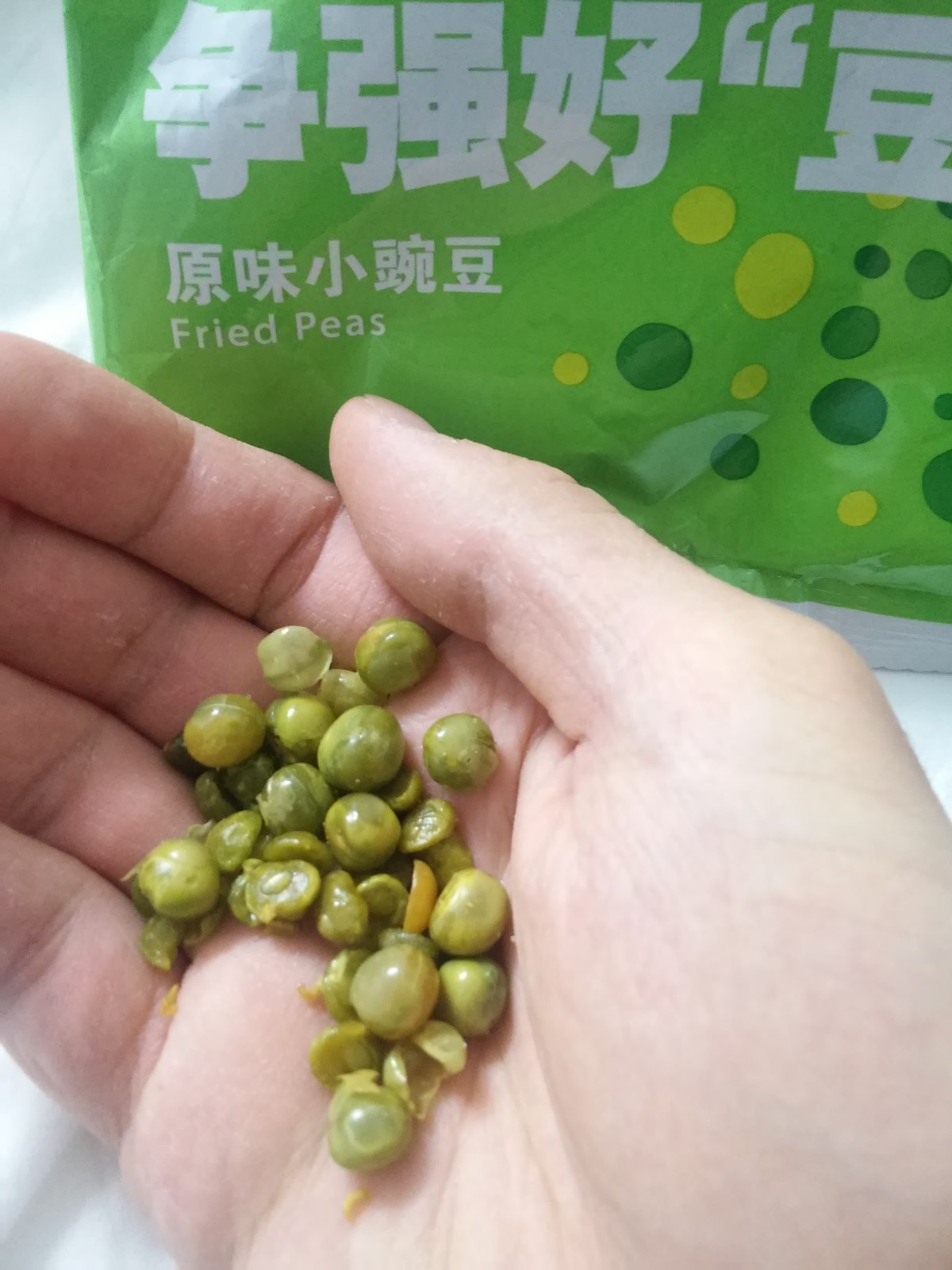This is a detailed color photograph, vertically oriented, featuring a close-up of a right hand holding several green and slightly yellowish fried peas. The hand, light brown in color, is cropped just below the fingers, extending from the bottom right corner to the mid-top section of the image. In the background, a bright green plastic bag with distinctive designs and text appears; the bag is adorned with darker green and yellow circles. The top of the bag displays Chinese characters, followed by Korean characters, and beneath them, in white text, it reads "fried peas." The snapshot captures the essence of someone showcasing the contents of the bag in their hand, highlighting the vibrant color contrast between the hand, the peas, and the packaging.